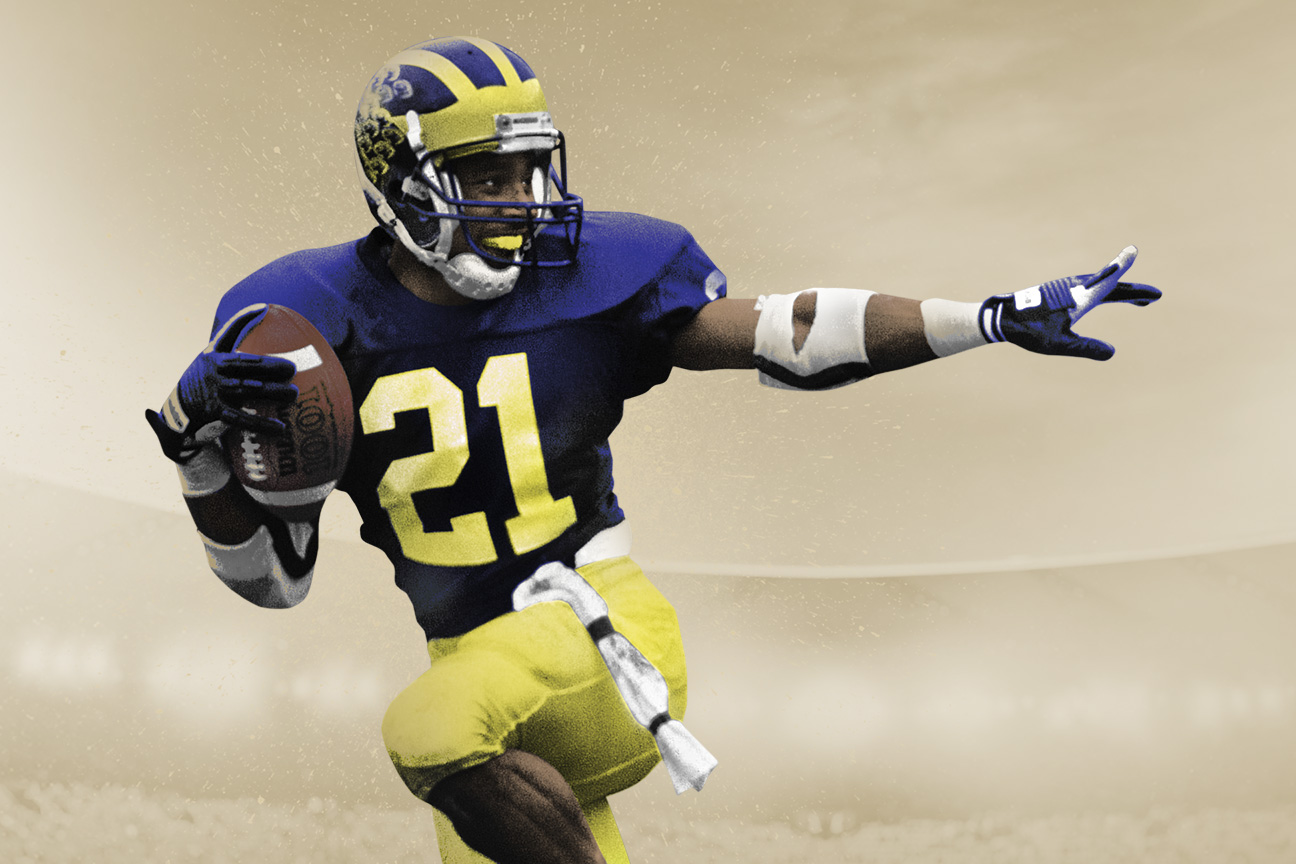This detailed, close-up photograph features an African American football player who is posed in a dynamic stance reminiscent of the Heisman Trophy posture. He is wearing a Michigan Wolverines college football jersey, identifiable by its navy blue color with yellow outlines and the number 21 emblazoned in gold on his chest. His right hand cradles a football against his right shoulder, while his left hand is extended as if he's about to deliver a stiff arm. The player’s left foot is in the air, indicating he is in motion, running to his left.

The football player’s expression is one of happiness, and he appears to be in his early 30s. He is equipped with a yellow, bright mouthguard and donning a purple and yellow helmet. His gloves are black, blue, and white, secured with Velcro. He stands against an off-white, beige-brown background. This image captures the player mid-action with great detail, highlighting his vibrant uniform and dynamic posture.